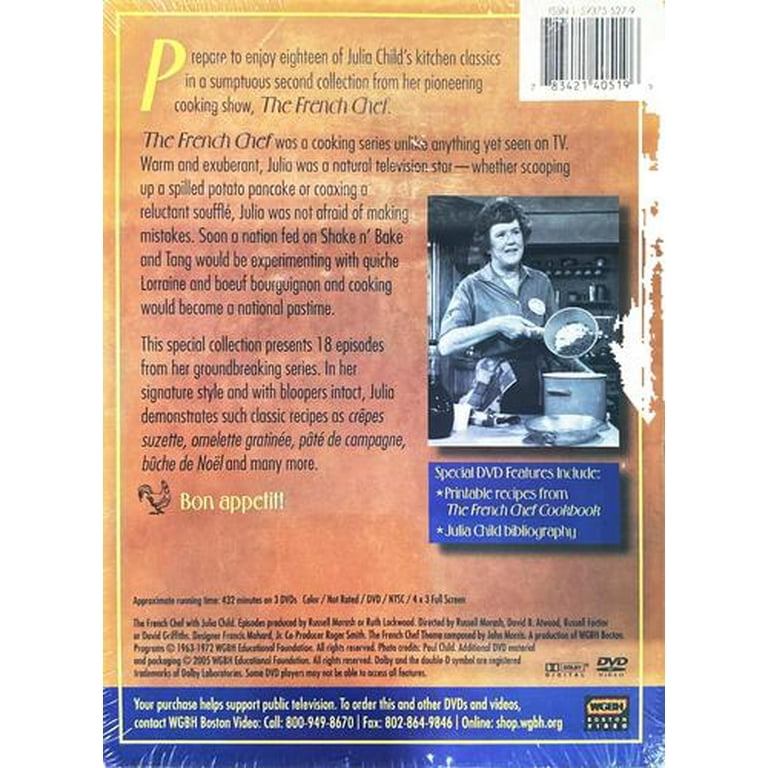The back of the DVD case for Julia Child's groundbreaking cooking series, "The French Chef," features a detailed and engaging layout. The top right showcases standard identifiers like the ISBN and scanning code. Prominently, the left side of the case includes a thorough description of the DVD's contents, highlighting "The French Chef" in bolded text. Below, it proudly markets special features such as printable recipes from "The French Chef" cookbook and a Julia Child bibliography.

A black and white photograph of Julia Child occupies the right middle section, displaying her in action as she cooks in a kitchen, holding a pan and ready to transfer its contents into a larger pot, surrounded by additional kitchenware. 

The description elaborates on the series, inviting viewers to savor 18 episodes of Julia Child's kitchen classics from her pioneering show. Julia's warm and exuberant personality shines through as she fearlessly navigates kitchen mishaps, transforming cooking into a beloved national pastime. Signature recipes demonstrated by Julia include Crêpe Suzette, Omelette Gratinée, Pâté de Campagne, and Bûche de Noël, all with her characteristic charm and unpolished authenticity intact.

The visual design includes a brownish background with a thin yellow border around the edges and a blue bottom section. A striking black rooster and the phrase "Bon Appétit" in yellow lettering add to the visual appeal. The bottom of the case contains finer details such as the running time of 432 minutes, pertinent copyright information, ordering details, and logos supporting public television, notably WGBH Boston Video and the DVD logo.